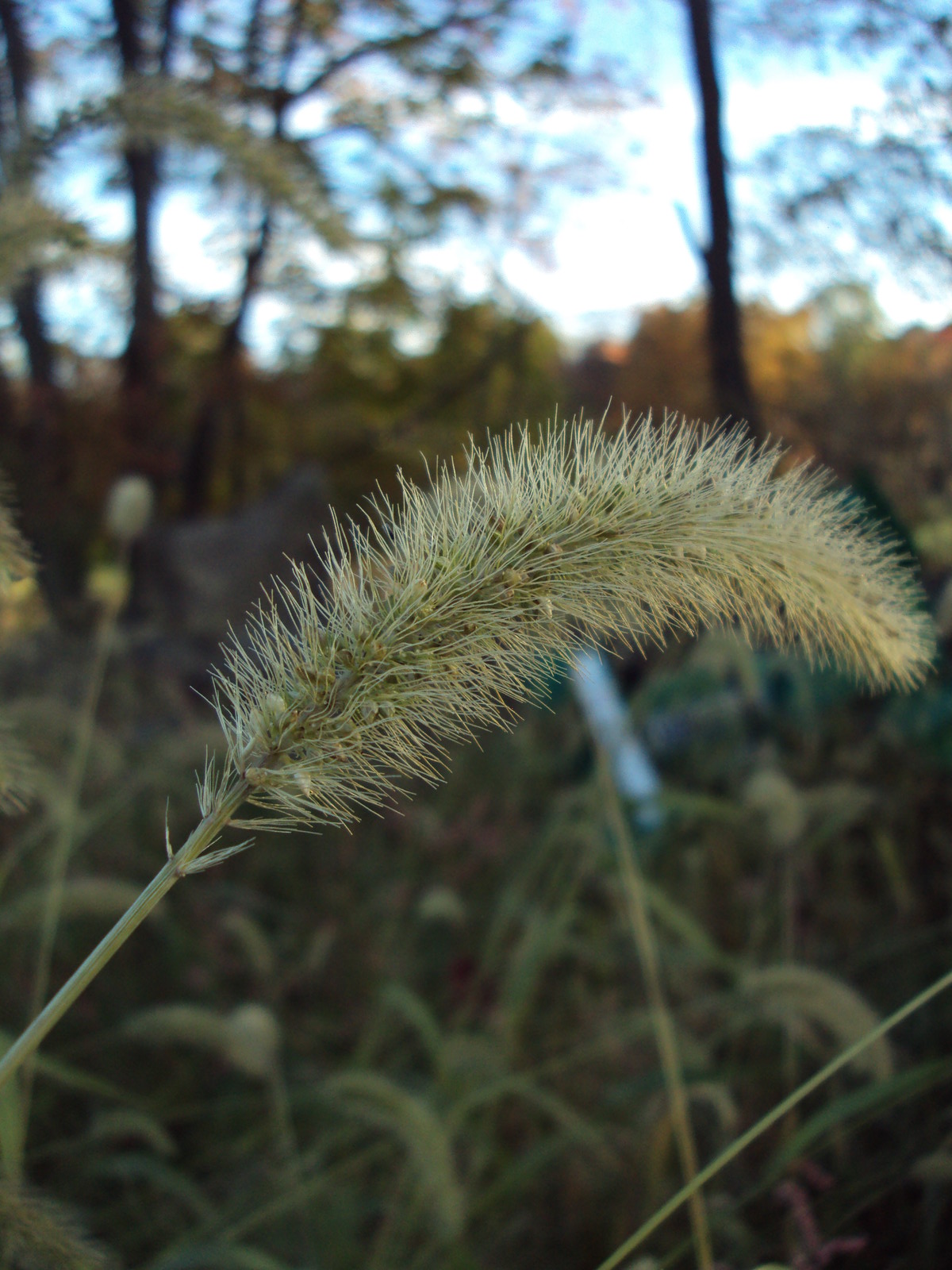In the image, we observe a field or a part of the jungle with a prominent plant in the foreground. The plant resembles a wheat plant, characterized by a single green stem and branches, adorned with a flower that has fine, thin petals. The flower is predominantly green with hints of yellow, and its pollen or seeds are also green and yellow. The background, although blurry, reveals various other plants, including thin trees and bushes with green, yellow, and red foliage. Amidst the slightly obscured scenery, additional tall trees can be discerned, suggesting a sunny and clear day.